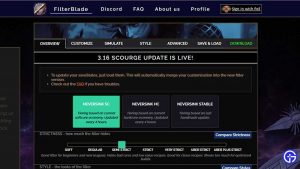The image is a pixelated, small screenshot of a computer software interface, which is challenging to discern in its entirety. The central feature is a webpage titled 'Filter Blade,' which is one of five primary tabs. The visible tabs include 'Filter Blade,' 'Discord,' 'FAQ' (Frequently Asked Questions), 'About Us,' and 'Profile,' with the 'Filter Blade' tab currently active.

The Filter Blade page appears to be related to some form of update or functionality within the software, specifically mentioning a "3.16 Scourge update is live!" There are additional sub-tabs on this page, labeled 'Delivery,' 'Style,' and more, which are not fully visible or clear. Within the main window of the 'Filter Blade' page, there seems to be a bar chart featuring a prominent green bar, although the precise details and text are difficult to read due to the image quality.

There is also a hint of another window partially visible off-screen, suggesting the presence of a multi-window interface within the software. The 'Discord' tab seems to point to a social or media source, though it’s not explicitly clear how it functions within this context.